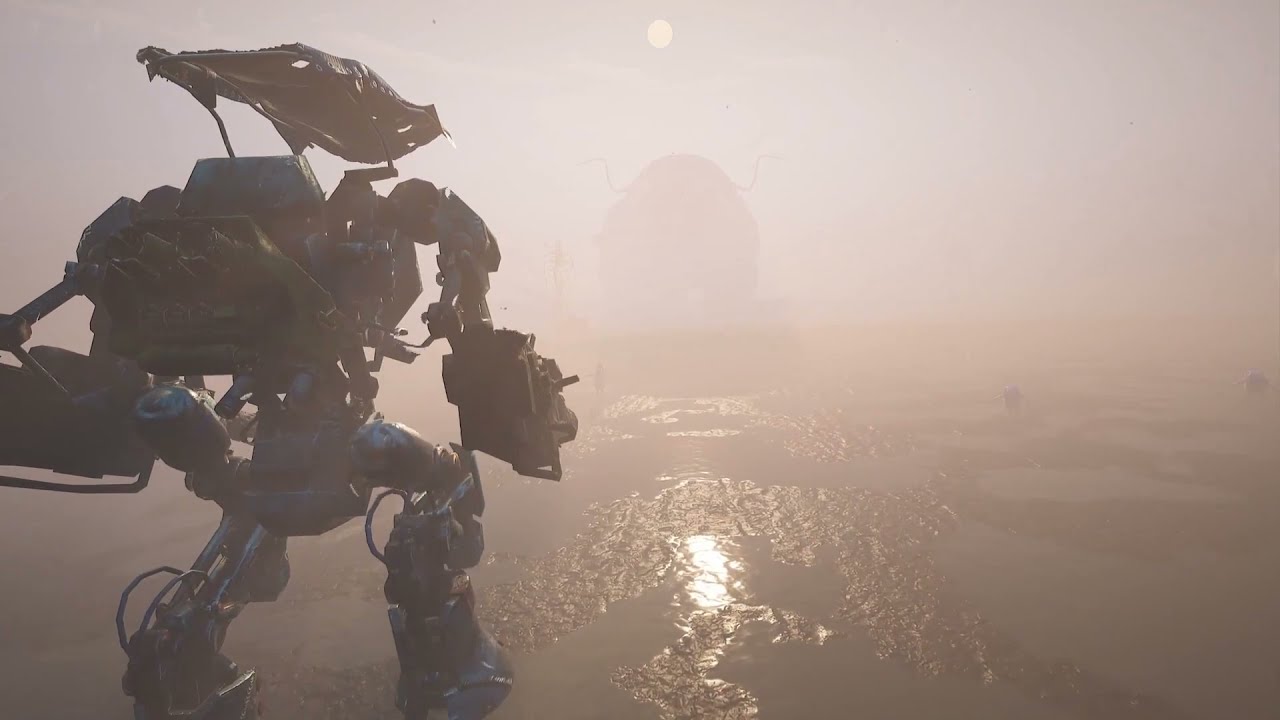The image is a detailed screen grab from a video game, showcasing a massive, heavily-armed mecha, which is a giant, human-piloted robot. Dominating the left side of the image, the mecha stands tall with visible cannons attached to its arms and legs equipped with a sophisticated hydraulic system, hinting at its advanced mechanics and combat readiness. Predominantly blue with a silvery hue, the mecha also displays an open hatch at the top, suggesting the pilot's possible exposure. The scene is enveloped in haze, casting a mysterious aura over the sandy landscape that appears wet in some areas, indicative of reflections suggesting nearby water. In the background, a large, indistinct, round object looms within the mist, possibly a celestial body such as the sun or moon, creating a focal point in the distance. Thin wires are seen trailing from the back of the mecha, enhancing its mechanical intricacy. The overall atmosphere is one of desolation and uncertainty, amplified by the hazy, ethereal quality of the setting.